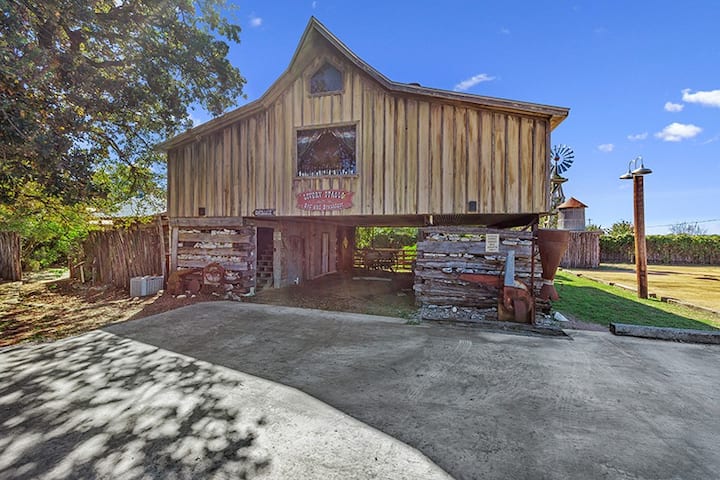The image depicts a two-story barn-like building situated on a well-manicured property with a bright blue sky dotted with scattered clouds as the backdrop. The structure's upper section is made of thin, vertical, light wooden planks reminiscent of a cabin, complemented by rough, horizontal wooden planks on the bottom, which resemble pallet wood and give the appearance of an old-school facility. The building includes a red sign with white letters that is difficult to read and features a square picture whose details are obscured by distance. In the background, a silo and a windmill are visible, hinting at this being a working farm. The left side of the image shows a tree with leafy yet open sections. The property includes a neatly paved driveway and expansive lawn, with some rusted machinery off to the side, suggesting it may also serve as a workshop or stables. Additionally, there is a small lamp at the front of the building, enhancing the rustic farm aesthetic.